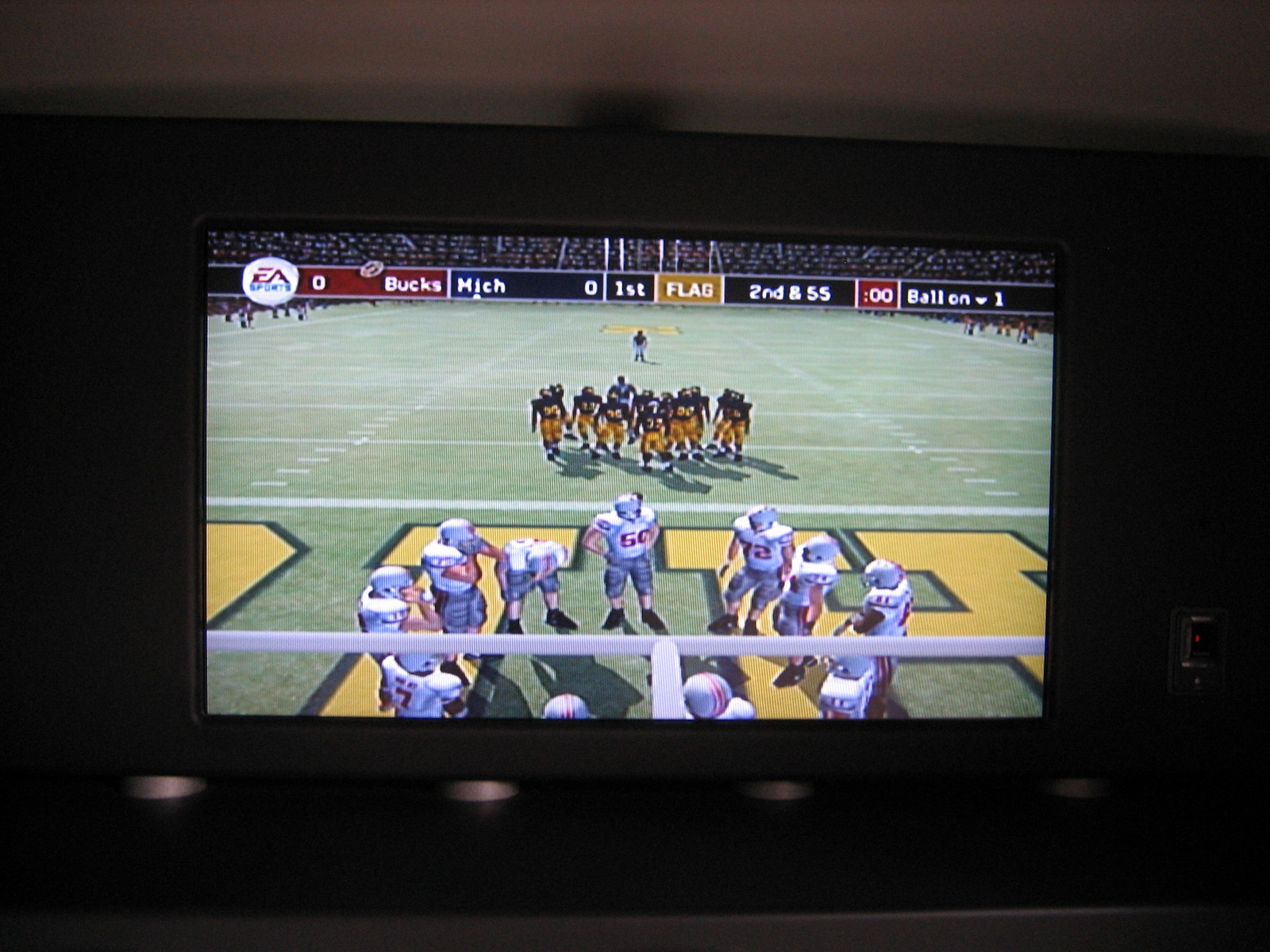The image depicts a dark room with a flat-screen TV mounted on a white wall, the only light emanating from the TV itself. The TV, sitting on four small silver circular stands on a black surface, is broadcasting a football video game. The screen shows a match between Ohio State and Michigan, with both teams clearly distinguished by their uniforms: Ohio State players are dressed in black and yellow, while Michigan players are in white and grey. The score is 0-0, and the game is in the first quarter with a second down and 55 yards to go. In the background, a virtual stadium is visible, filled with a simulated crowd. The on-screen interface includes a scoreboard that features the EA Sports logo in a white circle with blue text, various team statistics, and game information. The TV setup also includes a black and silver outlet with a switch on the right side, highlighted by a red indicator light.